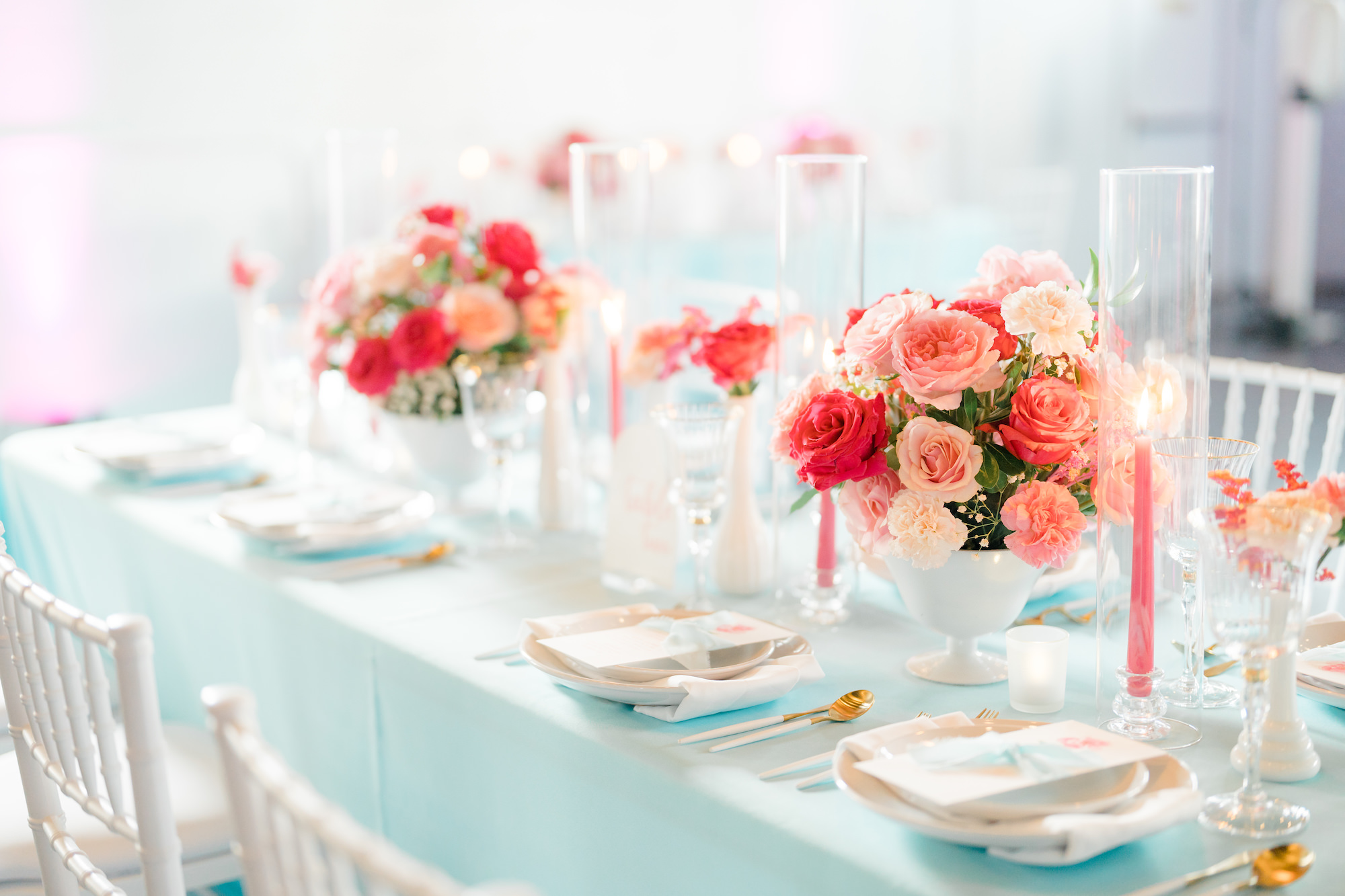A beautifully set dinner table is adorned with an array of vibrant flowers, featuring pink and red roses in both large and small white vases. The table is covered with a baby blue tablecloth that adds a touch of elegance to the setting. Long, pink candles are placed in glass flutes to protect the flames, enhancing the ambiance. Gold utensils with white handles are neatly arranged alongside plates that hold welcome or thank-you cards. The table is surrounded by white chairs, suggesting a special event such as a wedding or a birthday celebration. The overall setup is clean and sophisticated, with a bright and inviting springtime feel.